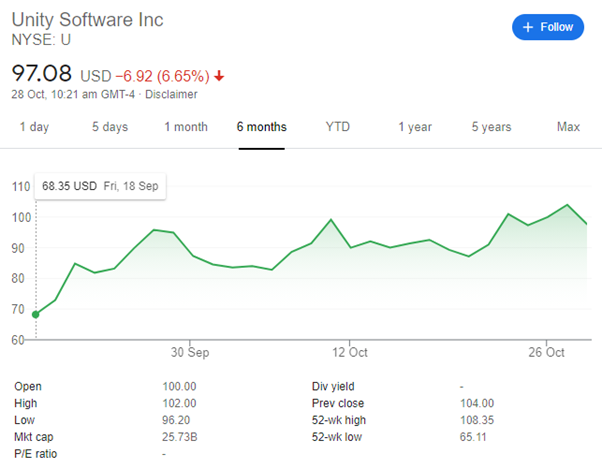In this image, we are looking at a screenshot displaying financial information in a graphical format. In the upper right corner, there is a "Plus Follow" button. Starting from the upper left, the display shows details related to Unity Software, Inc. traded on the NYSE under the ticker symbol 'U'. Below the company name, it lists significant financial data: the current stock price at 97.08 USD, a decrease of 6.92 USD or down 6.65%. The date mentioned is October 28th, and the current time is 10:21 AM GMT.

The graph depicted spans vertically from 60 to 110, with the horizontal axis covering dates from September 30th to October 26th. Beneath the graph, additional financial statistics are provided: the opening price at 100 USD, a high of 102 USD, a market capitalization of 25.73 billion USD, a previous closing price of 104 USD, a 52-week high of 108.35 USD, and a 52-week low of 65.11 USD.